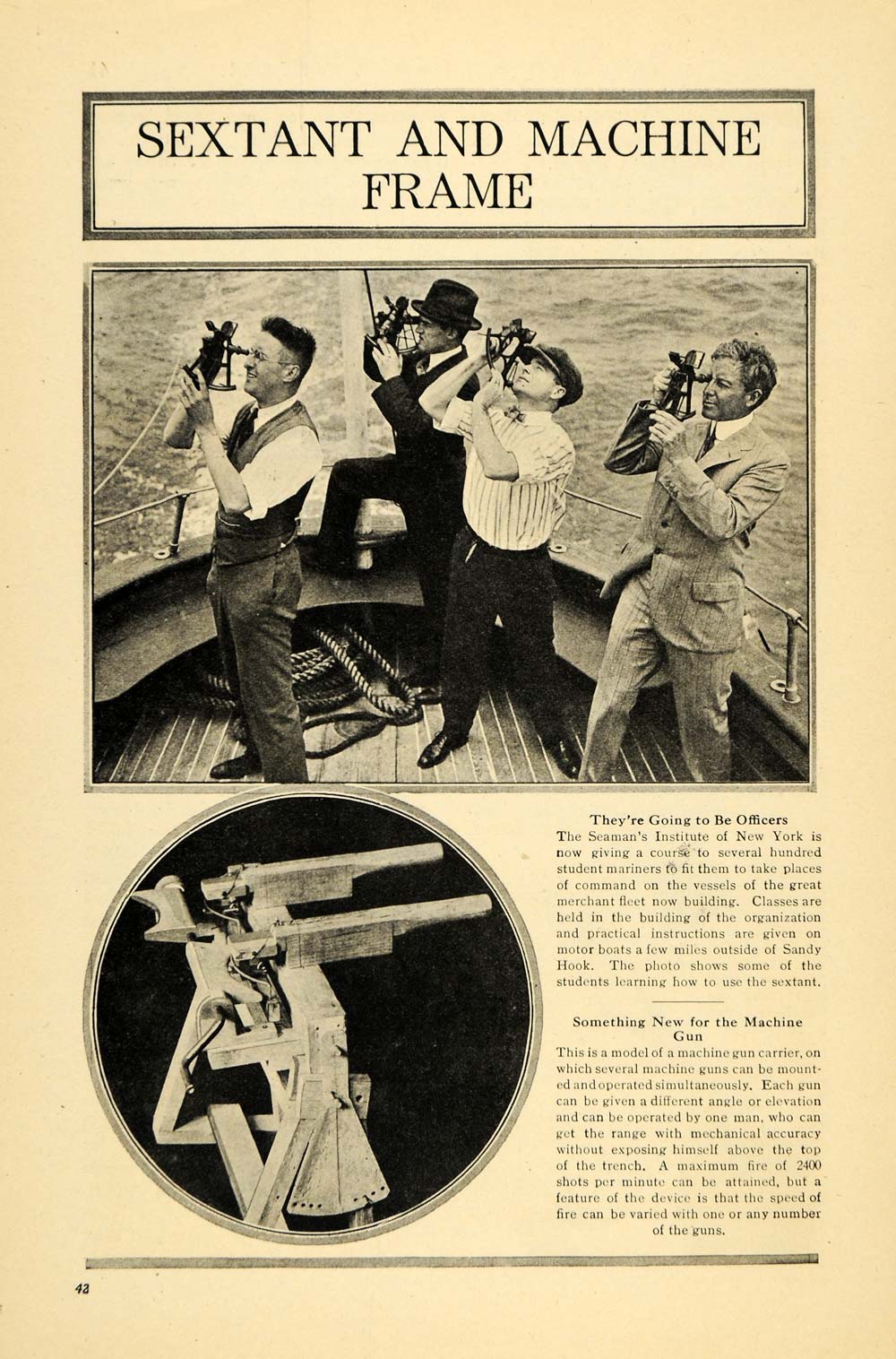This black-and-white image, taken from a very old newspaper clipping with a faded white or yellow background, features the headline "Sextant and Machine Frame" in bold black text at the top. Below this are four men standing on a boat, peering into the sky while handling what appears to be early, somewhat rudimentary cameras. The men, who are student mariners from the Siemens Institute of New York, are likely practicing the use of these devices as part of a training program designed to prepare them to become officers for the merchant fleet. A closer black circular inset shows a detailed view of the camera, which intriguingly resembles a machine gun carrier capable of mounting and simultaneously operating several machine guns, as described by its accompanying article. This article, with bold headlines, announces the innovative machine gun model and details the mariners' education, underscoring the practical training they receive. The overall composition of the image on the newspaper page gives a glimpse into historical maritime training and technological advancements in navigational and weaponry equipment.